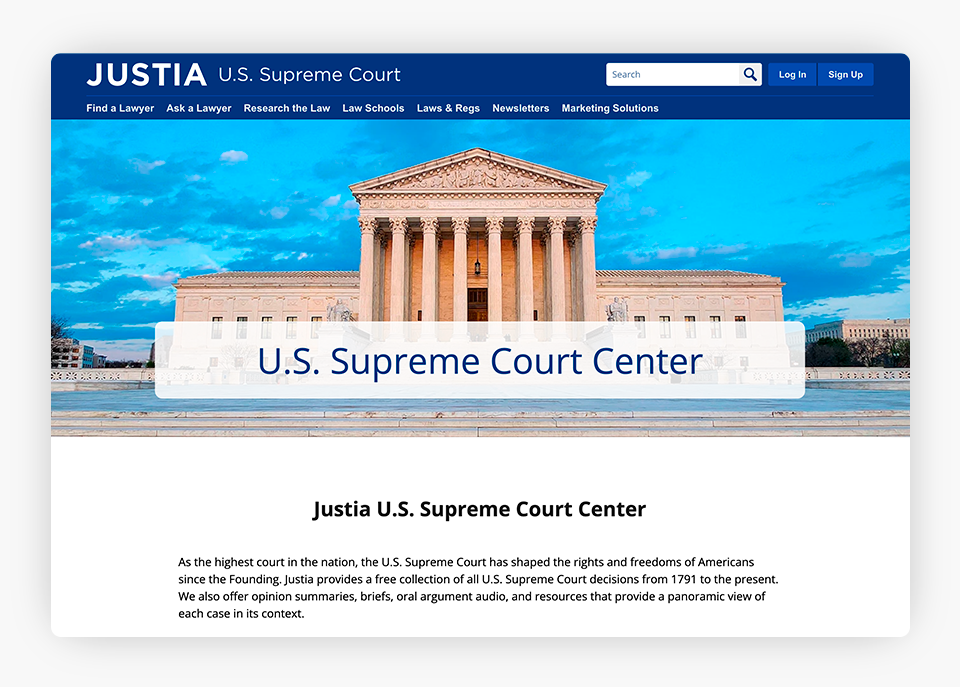This image is a screenshot of the Justia U.S. Supreme Court website, specifically the desktop version. The site features a clean, white background with a dark blue menu bar at the top. Prominently displayed in white lettering on the menu bar is the title "Justia U.S. Supreme Court." To the right of this title, there is a search box iconified by a magnifying glass, followed by lighter blue buttons labeled "Log In" and "Sign Up."

Below this menu bar, a secondary navigation menu offers links to various sections of the site in white text against the lighter blue buttons. These sections include "Find a Lawyer," "Ask a Lawyer," "Research the Law," "Law Schools," "Laws and Regs," "Newsletters," and "Marketing Solutions."

Central to the screenshot is an image of the U.S. Supreme Court building. The building is depicted in a very light tan color, featuring multiple iconic columns at its front. The architectural form is square, with a prominent, slanted A-frame roof crowning the middle section. Directly beneath this image, the text "U.S. Supreme Court Center" is presented in blue, followed by a black text block stating "Justia U.S. Supreme Court Center."

The detailed caption continues to explain the significance of the U.S. Supreme Court, noting that, as the highest court in the nation, it has played a critical role in shaping the rights and freedoms of Americans since the founding of the country. The description highlights the resources provided by Justia, which include a free collection of all U.S. Supreme Court decisions from 1791 to the present, alongside opinion summaries, briefs, oral argument audio, and additional resources that offer a panoramic view of each case in its context.